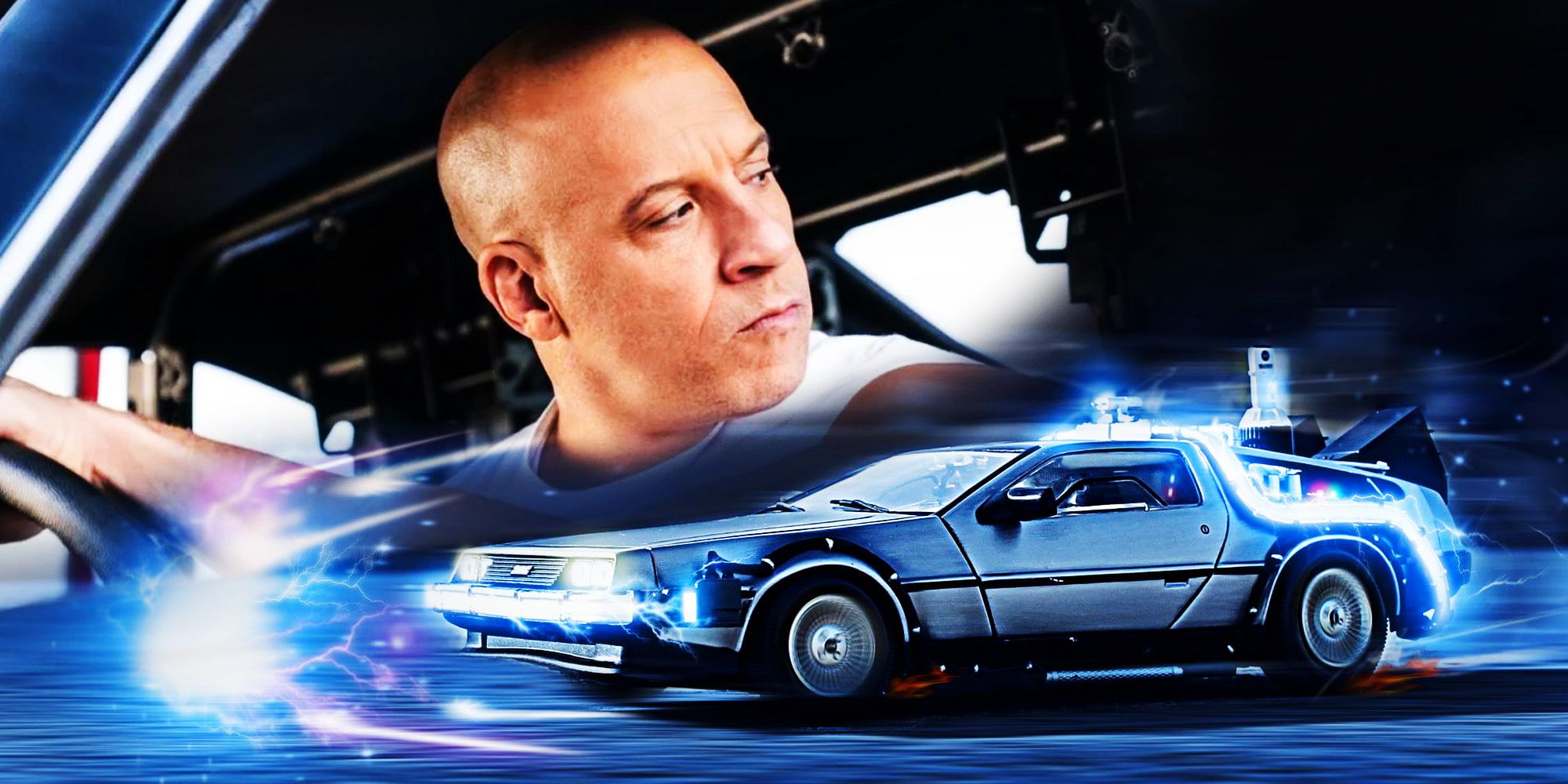In this detailed composite image, the top section features a zoomed-in view of Vin Diesel as his character Dom Toretto from the Fast and Furious franchise. Dom, with his signature bald head, has his hands on the steering wheel and is looking back over his left shoulder with a concentrated expression, emphasizing an aura of determination. His presence appears as if he's in the act of driving a car, seamlessly integrated into the scene. Below him, the iconic DeLorean from the Back to the Future series speeds to the left, enveloped in a distinctive aura of blue electricity and sparks, symbolizing its time-travel capabilities. The DeLorean is showcased with striking detail, from its silver body to the absence of its characteristic gull-wing doors, further blending the two film worlds. The car's motion is accentuated by the surrounding lightning and force field effects, set against a darker, dramatic background that underscores the image's electrifying and fantastical nature. This mash-up creatively contrasts the high-octane world of Fast and Furious with the sci-fi brilliance of Back to the Future.